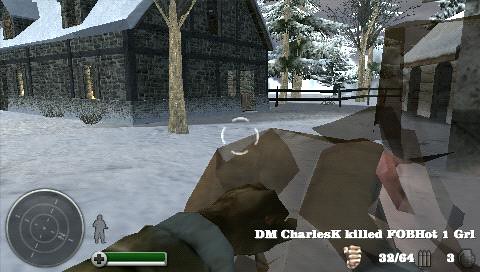In this detailed video game scene, an outdoor snowy environment unfolds in front of the player. To the left, there's a gray brick building with a triangular roof blanketed in white snow. A leafless tree stands in front of the house, and more snow-covered pine trees are visible in the background, enhancing the wintry setting. On the right side, part of a tan building with arched dark doorways peeks into the frame, providing contrast to the gray structure. The bottom of the image features a first-person perspective, showing the character's hands—one clad in a black glove and the other wrapped in white bandages—gripping a brown object. A circular crosshair is centered on the screen, indicating the player's aim.

In the lower-left corner, a black circle resembling a compass serves as a scanner or map, with a green figure outline next to it, likely indicating the player's remaining lives. Below this, a green health bar, accompanied by a circle with a plus sign, displays the player's health status. On the bottom right, in white text, the game records, "DM Charles K killed FOB HOT 1 GRL." Additional game information includes an icon of a grenade with a count of three, and an ammo count reading "32/64." Ominously, in the distance, dark cloaked figures appear to be moving towards one of the buildings, adding an element of suspense to the scene. A fence separates the two structures, completing the immersive and detailed portrayal of this wintry gaming landscape.